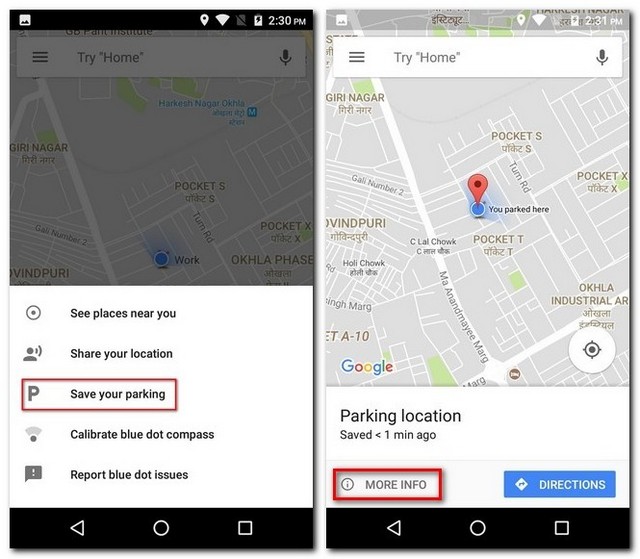This image showcases two smartphone screens displaying a tutorial for a map application. Both screens feature a search bar at the top labeled "home," with the prompt "Try 'home'" highlighted in gray and enclosed in quotation marks. 

The left screen displays a map with a grayed-out search box slightly lower than its counterpart on the right. Below the search bar on the left, a white box contains various options: "See places near you," "Share your location," and "Save your parking." Notably, the "Save your parking" option is distinguished with a red outline.

The right screen mirrors the left but shows the search box positioned slightly higher up on the interface, providing a closer view of the described features. 

Together, these screens provide step-by-step guidance on utilizing specific map app functionalities for location searches and parking features.